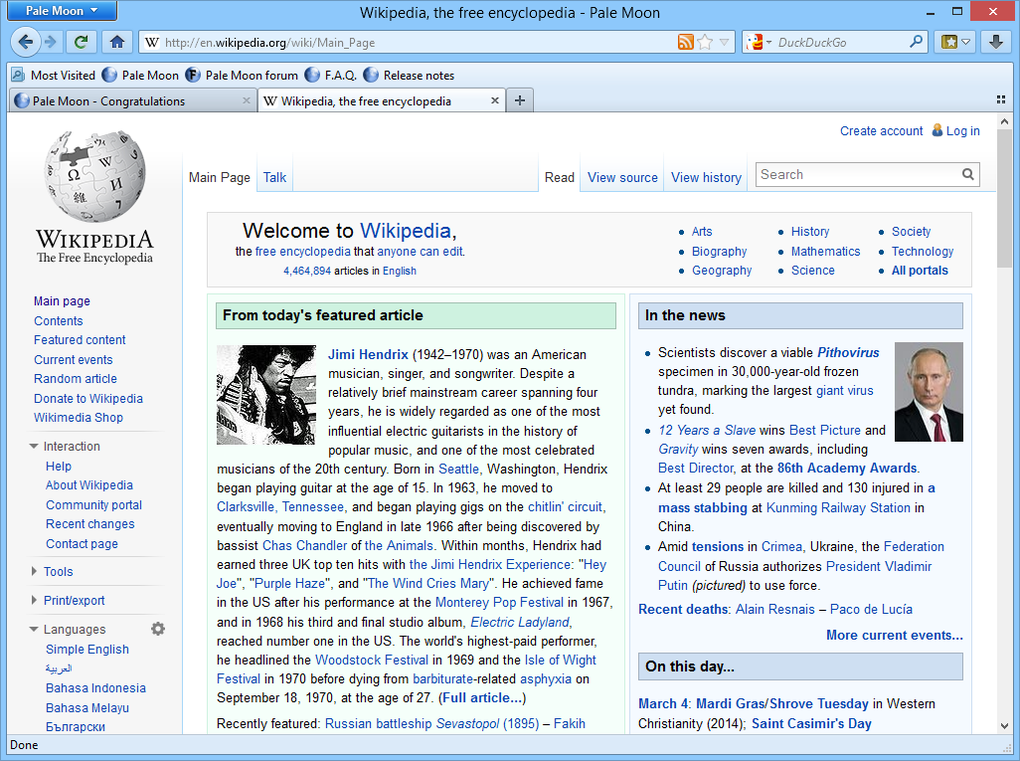The image features a screenshot of the Wikipedia homepage viewed on the Pale Moon web browser. At the top, a banner reads "Wikipedia, the free encyclopedia." Below, a search bar is prominently displayed, followed by a few frequently visited links labeled "Pale Moon," "Pale Moon forum," "FAC," and "Release note." The familiar Wikipedia tagline, "Welcome to Wikipedia, the free encyclopedia that anyone can edit," appears next, alongside various article categories such as Arts, History, Society, Biography, Mathematics, Technology, Geography, Science, and links to "All portals."

The left column features "From today's featured article," which highlights Jimi Hendrix, noting his birth and death years (1942-1970) and describing him as an American musician and singer. The right column, titled "Also in the news," mentions recent events including the discovery of a variable perthovirus, a film titled "12 Years a Slave," and a tragic update stating that at least 29 people have been killed and 130 injured.

The screenshot captures the essence of Wikipedia's homepage, showcasing both its informative content and its communal, open-editing spirit.